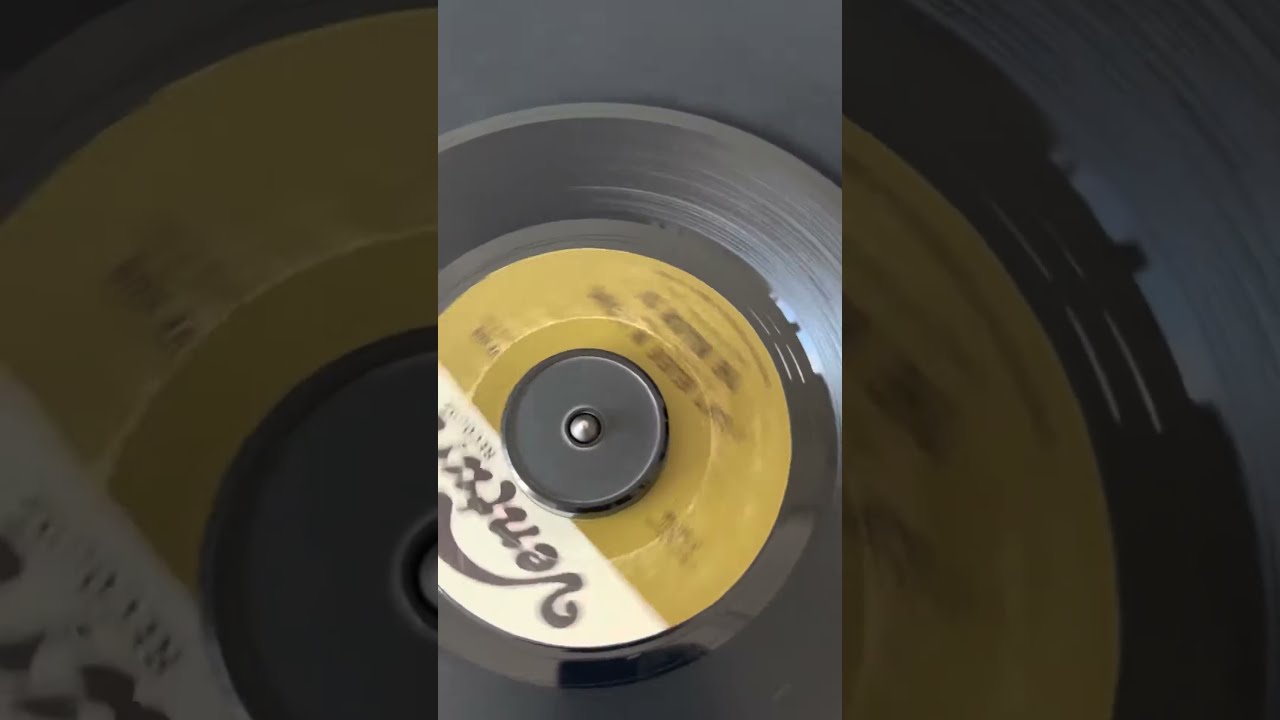The image showcases a close-up of a vinyl record, specifically focusing on its central label. The record, which appears to be in motion as evidenced by a slight blur, is a shiny black color with potential brown hues. The central label, which is partially zoomed in and darkened in the left and right thirds of the image, prominently displays the word "Venture" in a stylized, possibly 70s-inspired font, with the 'V' artistically curling over the subsequent letters. The top third of the label is white with a brown font, while the bottom third transitions to a golden-brown or butterscotch color. Surrounding the label, the vinyl's concentric circles and grooves are visible, signifying the areas where the record player’s arm would read the music. The center of the record features a plastic hub with a metallic component, essential for securing the record during playback. Further text, indicating song titles, is present but illegible due to the image's motion blur.